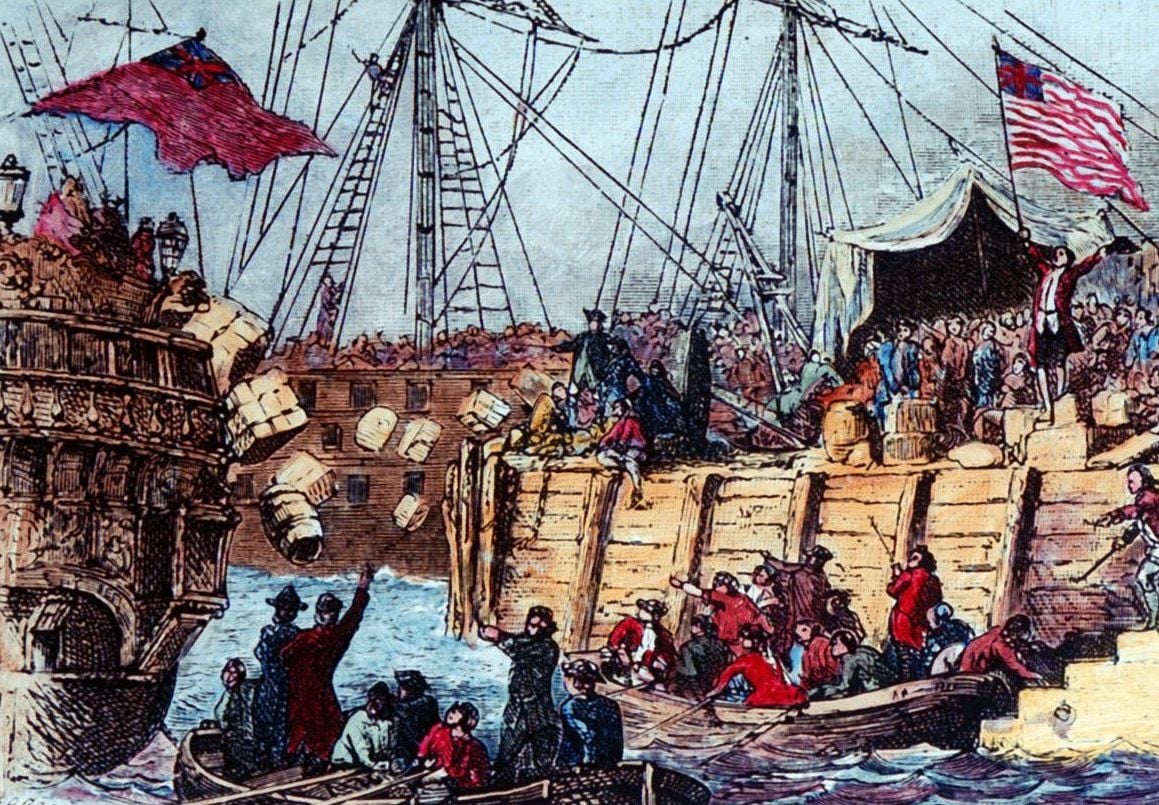This detailed hand-drawn, full-color illustration features a historical maritime scene that hints at the Boston Tea Party. The sky is gray, setting a somber tone above the bustling waters. Dominating the scene are three large, old-style wooden sailing ships, their sails furled and masts bristling with rope ladders and other naval architecture. Smaller rowboats are clustered around the ships, with figures actively rowing.

The deck of the largest ship is teeming with dozens of people, meticulously detailed. Their actions suggest the rampant disposal of tea into the water, with boxes and barrels being hurled overboard in a chaotic fashion. This scene is reminiscent of the Boston Tea Party, although some flags in the image are not historically accurate, featuring red crosses and variations of the American flag—with one flag showing a blue square with a red star and red stripes. There are people climbing stairs onto the vessels, enhancing the historical recreation's authenticity, despite the artistic liberties taken with the flags.

Overall, the illustration captures the energy and essence of a pivotal event in American history through detailed and vibrant artistic expression.